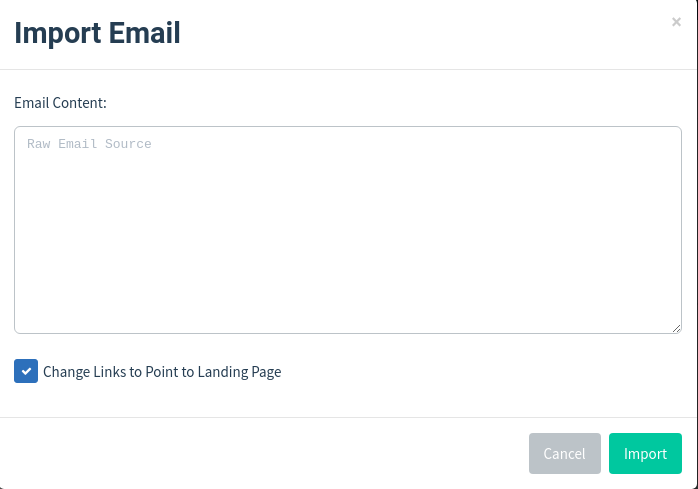This image is a screenshot of a user interface. At the top left corner, there is a label that reads "IMPORT EMAIL" in large, bold letters. Adjacent to this label, on the right side, is a faint gray X icon. A thin black vertical line runs along the right side of the image.

Beneath the "IMPORT EMAIL" heading, a thin gray horizontal line separates the upper section from the content below. Directly below this line, the text "Email Content" is displayed. Underneath this heading, a box bordered by a light gray trim contains the text "RAW EMAIL SOURCE" in large, bold, capital letters rendered in a light gray font.

Below the "RAW EMAIL SOURCE" box, on a white background, there is a blue box with a white check mark in its center. To the right of this blue box, a sentence reads "CHANGE LINKS TO POINT TO LANDING PAGE" in large, bold capital letters.